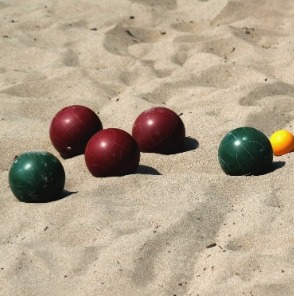This is a detailed square-format color photograph taken outdoors on a sunny day, with no visible border. The background is a light beige sandy surface with multiple imprints and small bits of debris, suggesting frequent disturbances by wind or foot traffic. The central focus of the image is six bocce balls, round and shiny, reflecting sunlight. Arranged on the sand, there are two dark green balls—one on the left and one on the right. Between them are three dark red balls. Additionally, there is a smaller yellow ball located behind and to the side of the green ball on the right. The balls are not perfectly aligned but appear to be interspersed throughout the sandy surface, creating a natural, yet organized composition. Lines and textures are visible on the green balls, adding to the realistic and representational quality of the photograph.